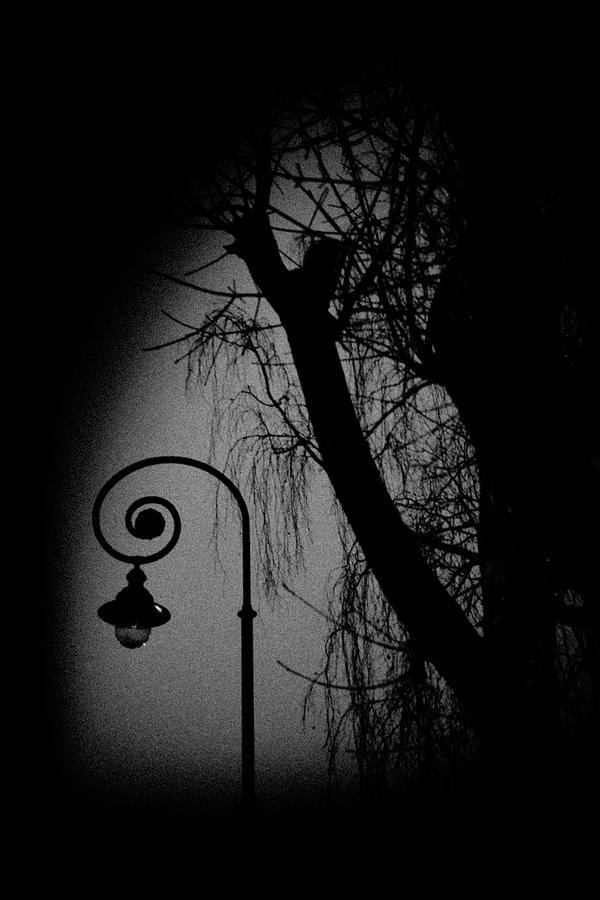This ominous black and white image, likely a photo or painting taken at night, features a central focus on a streetlight and a silhouetted tree. The streetlight pole emerges from the bottom and curves dramatically, forming a spiral pattern reminiscent of a snail shell. From the end of the curving pole hangs an unlit lamp, crafted in a delicate, bulbous shape, casting subtle highlights against the dark backdrop. In the background, a large tree trunk with spreading branches and twigs stretches upward, rendered in deep silhouette. The overall composition is set against an off-white to grayish background, starkly contrasting with the black silhouettes and evoking a haunting, nocturnal atmosphere. The edges of the image dissolve into complete darkness, further enhancing the night-time mystery and depth of the scene.